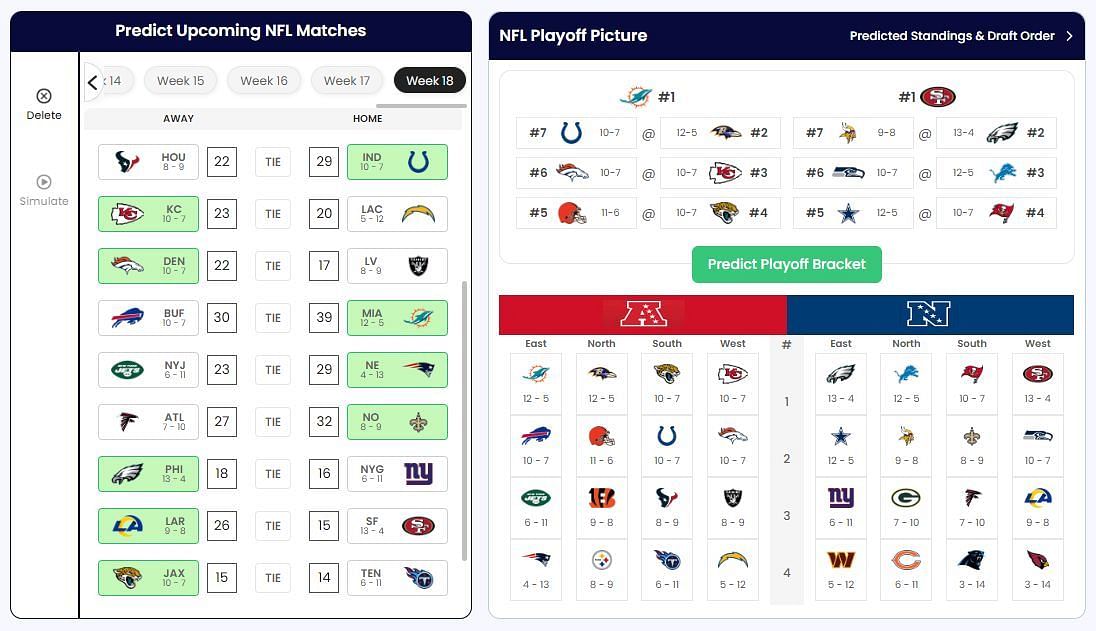This image showcases a detailed representation of a combined NBA and NFL playoff picture. The image is divided into two main sections. On the left, there is a section labeled "Predict Upcoming NFL Matches," featuring a top menu which allows users to select the week of interest; currently, it is set to Week 18. Below this menu, the section is organized into two columns headed 'Away' and 'Home.'

In the 'Away' column, the first item listed is the Houston Texans, displaying their logo along with the text "Houston 8-9" and a score of "22." Adjacent to this, in the center, it says "Tie" alongside a score of "29," indicating a match result. 

In the 'Home' column to the right, it lists "Indy 10-7," referring to the Indianapolis Colts with their respective season record. 

On the right side of the image, there are additional details presumably related to the NBA and NFL playoff scenarios, although specific scores are mentioned without further context. The overall layout and captions allow for interpreting detailed playoff predictions and match results, helping fans anticipate and analyze the outcomes of future games.